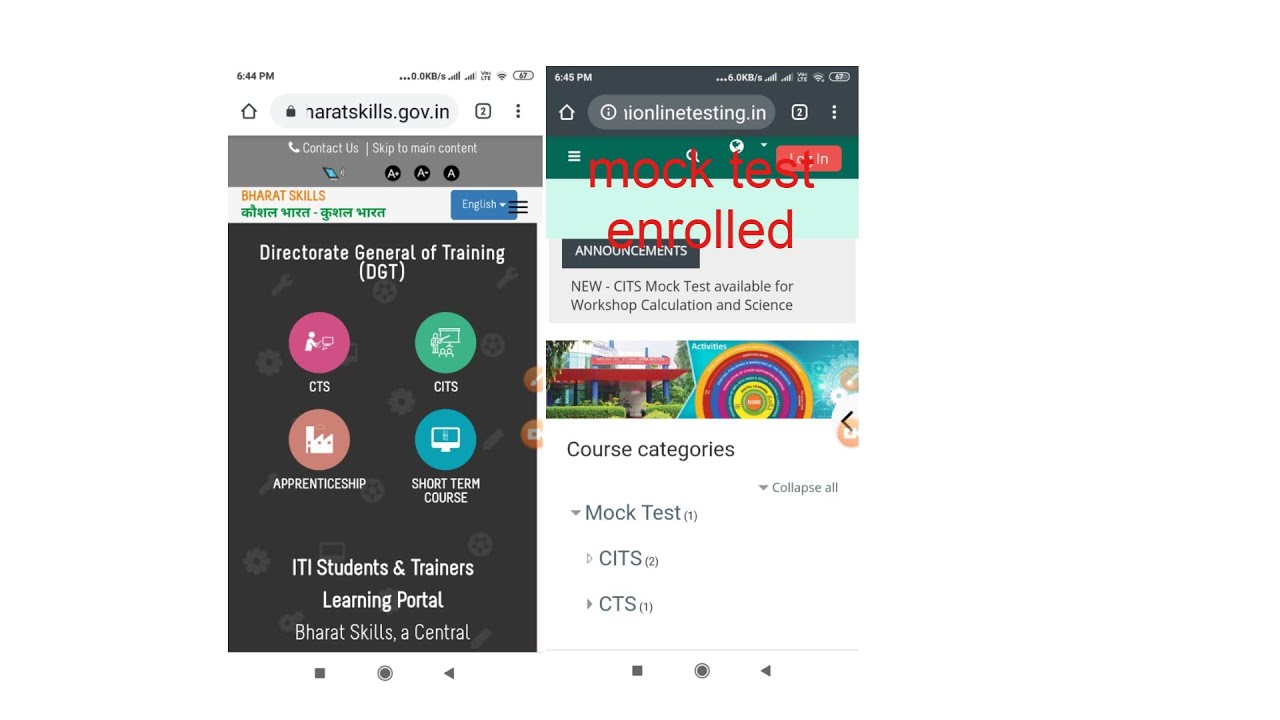**Caption:**

The attached images display two sequential screenshots from the Directorate General of Training (DGT) ITI Students and Trainers Learning Portal, taken a minute apart at 6:44 p.m. and 6:45 p.m., respectively.

In the first screenshot, timestamped at 6:44 p.m., the interface is predominantly gray. The section highlights various educational programs: 'CTS' inside a pink circle, 'CITS' within a green circle, 'Apprenticeship' in a reddish off-red circle, and 'Short-Term Courses' in a blue circle. The banner prominently features the portal's name, "ITI Students and Trainers Learning Portal," and includes the "Bharat Skills" initiative.

The second screenshot, timestamped at 6:45 p.m., shifts to highlight the portal's functionalities and updates. Notably, there are icons and details for "Mock Tests" and "Road Announcements." A new notification mentions the availability of new CITS mock tests for 'Workshop Calculation and Science.' Below is the 'Course Categories' section, listing various mock test subjects: 'CITS' with (1), 'CTS' with (2), and another CTS also labeled with (1). At the very top, the login button is prominently displayed in white text on a red rectangular background, facilitating access to the platform for registered users.